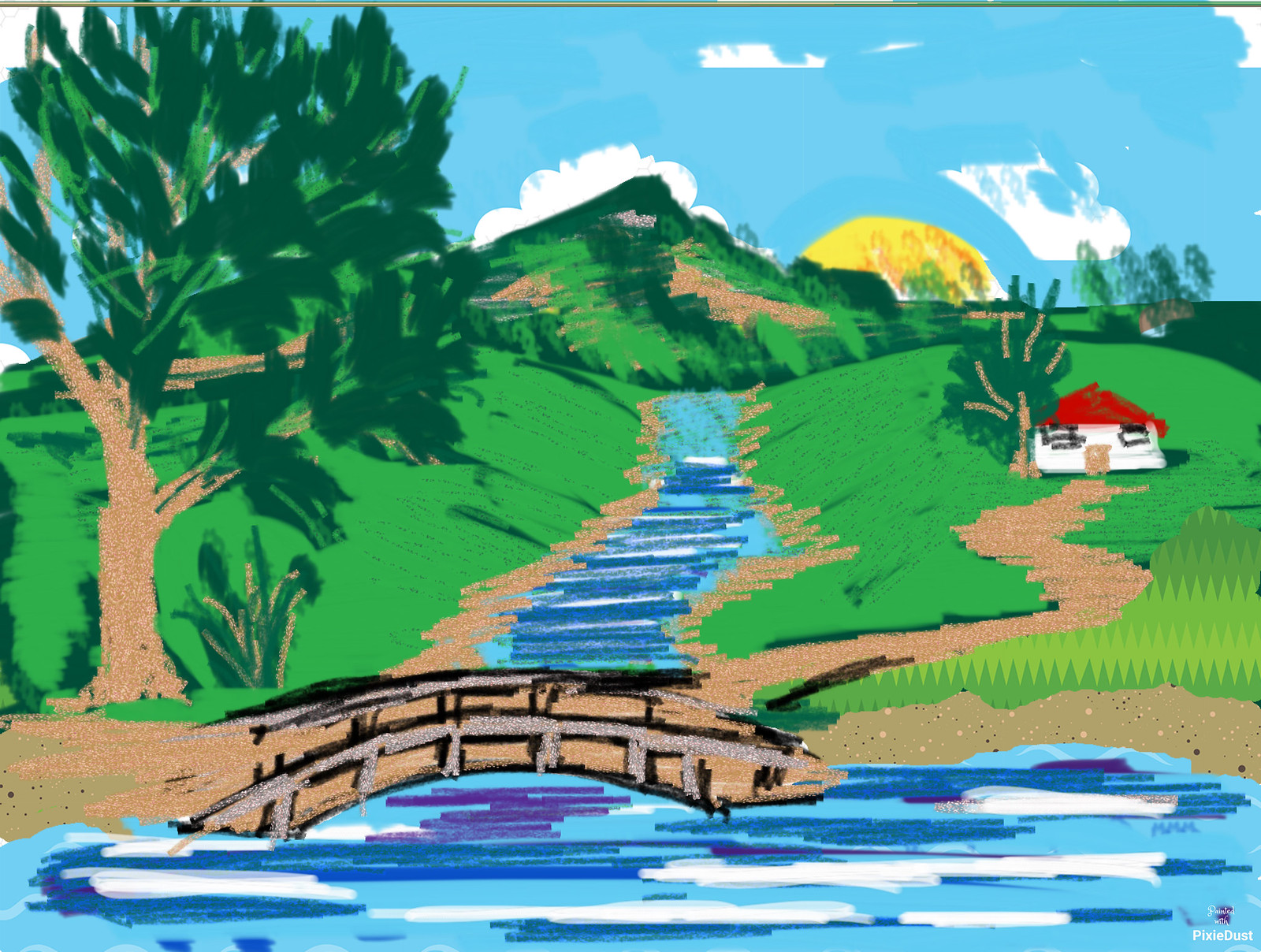This vibrant, pastel chalk-style digital artwork, possibly created in a program like Microsoft Paint, portrays a serene landscape under a bright blue sky dotted with fluffy white clouds. A green mountain, tinged with patches of brown soil, dominates the background, with the setting sun casting a warm glow to the right. A stream flows from the middle of the mountain towards the foreground, passing under a gracefully curved Japanese-style bridge, with blue water rippling gently beneath it. To the right of the bridge stands a quaint white house with a red roof, tucked away near a large tree. The tree, positioned to the left and closer to the viewer, adds depth to the scene. Additional smaller trees dot a rolling field behind the house. The text "pixie dust" is inscribed at the bottom right, hinting at a whimsical touch in the art.